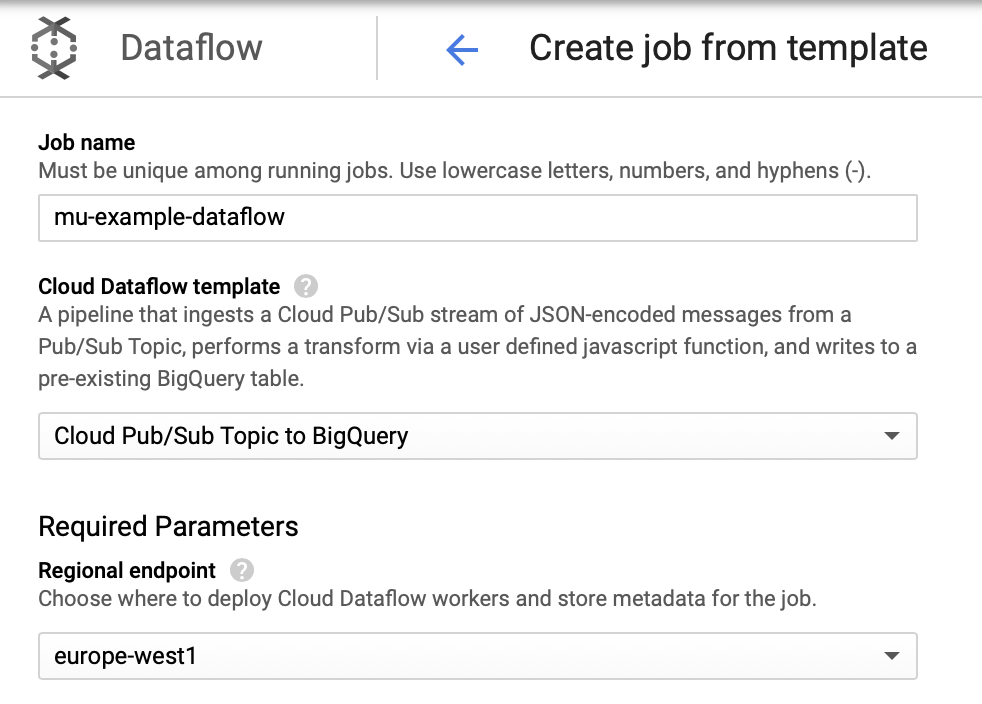The image appears to be a screenshot taken from a computer or smartphone device, displaying a user interface with no distinct background color, utilizing the default white background. At the top of the image, there is a gray ombre horizontal bar transitioning from gray to white. On the upper left-hand side of this bar, there is a gray icon followed by the text "Data Flow," separated by a short thin gray line.

Moving down, there is a blue arrow pointing to the left, adjacent to black text that reads "Create Job from Template," followed by another thin separating line. Below this section, on the left-hand side, the text "Job Name" is displayed in bold black font. Underneath, less bold text explains that the job name must be unique among running jobs and should only use lowercase letters, numbers, and hyphens. Beneath this text, there is a long input box where users can enter the job name, with a provided example.

Further down, in bold black, the text "Cloud Data Flow Template" is displayed, accompanied by a small question mark icon that provides additional information upon interaction. Below this section, there is another long rectangular input box with a dropdown arrow, allowing users to select a template. The current selection within this box is "Cloud Pub/Sub Topic to BigQuery."

Lastly, the text "Required Parameters" and "Regional Endpoint" are shown in bold black font, with another question mark icon providing further description. The description explains that users should choose a regional endpoint to deploy Cloud Data Flow workers and store metadata for the job. The current selection is "europe-west1," with an associated dropdown arrow for changing the region.